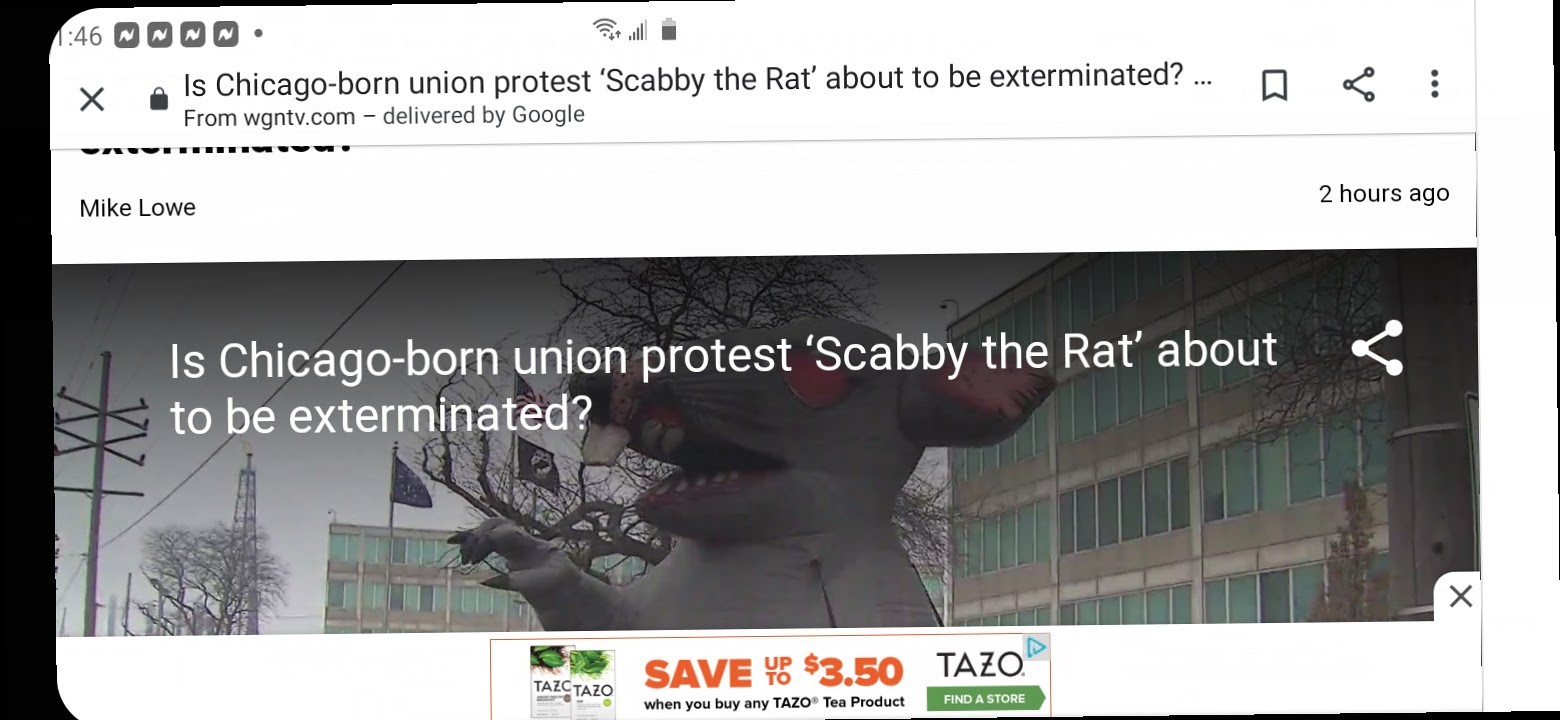The image captures a rectangular screenshot from a digital device, likely a phone, characterized by a pronounced black border around the image which tilts slightly left, exposing a broader black margin on the left side. At the top of the screen, in a white header, the time is displayed as 1:46, alongside icons for Wi-Fi, battery, and reception, hinting that it is a phone screen. Below this, there's an address bar reading, "Is Chicago-born union protest Scabby the Rat about to be exterminated from WGNTV.com delivered by Google," followed by the name "Mike Lowe" and a timestamp indicating "Two hours ago." 

Prominently, the image features a large inflatable rat sculpture with menacing red eyes, sharp teeth, and claws, set against a backdrop of office buildings under a dark gray sky intertwined with telephone poles. Overlaid on the photograph is the text, "Is Chicago-born union protest Scabby the Rat about to be exterminated?" Towards the bottom, there's an advertisement for Tazo Tea, highlighted in orange and black text, indicating a saving of up to $3.50 on any Tazo Tea product, accompanied by a green banner urging to "Tazo find a store."